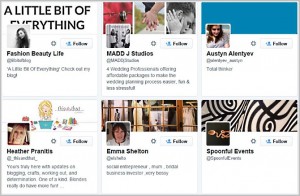The image depicts a small screenshot of a website or social media platform, likely Twitter. It showcases a layout consisting of a larger rectangle divided into six smaller squares, each containing different items and bordered neatly. The top left panel features a banner with the text "A Little Bit of Everything," with categories listed beneath like "Fashion," "Beauty," and "Life," alongside a picture of a young woman with long hair.

Adjacent to this, on the right side, is the profile for 'Magi Studios,’ which includes three header images: one of a bird, another of people holding hands, and a third of two people kissing. Below this header, the name 'Austin Magentavive' appears, accompanied by a profile picture of a woman framed by a blue top panel.

In the second row, the first panel features 'Heather Prentice,' showcasing a cartoon graphic of a woman engaged in various activities. Next to that is 'Emma Shelton,’ whose profile picture captures her looking forward, with what appears to be French doors or windows visible in the background, suggesting an outdoor scene.

The last panel in the row features 'Spoonful Events,' with an op-art inspired design at the top. The interface also includes follow icons, typical of Twitter, corroborating the screenshot’s social media origin.